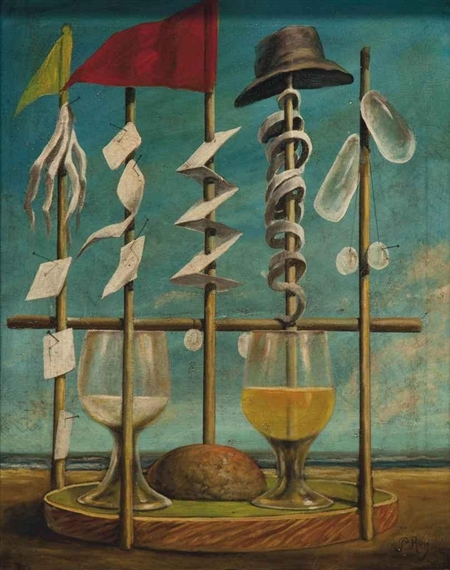The painting presents a surreal, abstract scene that feels almost like a visual puzzle. Central to the composition is a round, green wooden platter with a brown rim, set against a backdrop that suggests a beach with an ocean in the distance. Atop the platter rests a loaf of bread, accompanied by two goblets—one containing a yellowish liquid and the other a whitish liquid. Surrounding the platter are five wooden poles, each adorned with peculiar objects. One pole features a hat perched on top and what appears to be a snake coiled around it. Another holds two milk bottles and marbles. There are also poles with red and green banners, as well as pieces of folded paper affixed to them. The use of colors such as blue, yellow, red, black, white, and golden adds to the enigmatic nature of the scene. The entire composition evokes a sense of aged mystery, combining the aesthetics of surrealist and possibly ancient art, hinting at some deeper, perhaps symbolic, meaning.